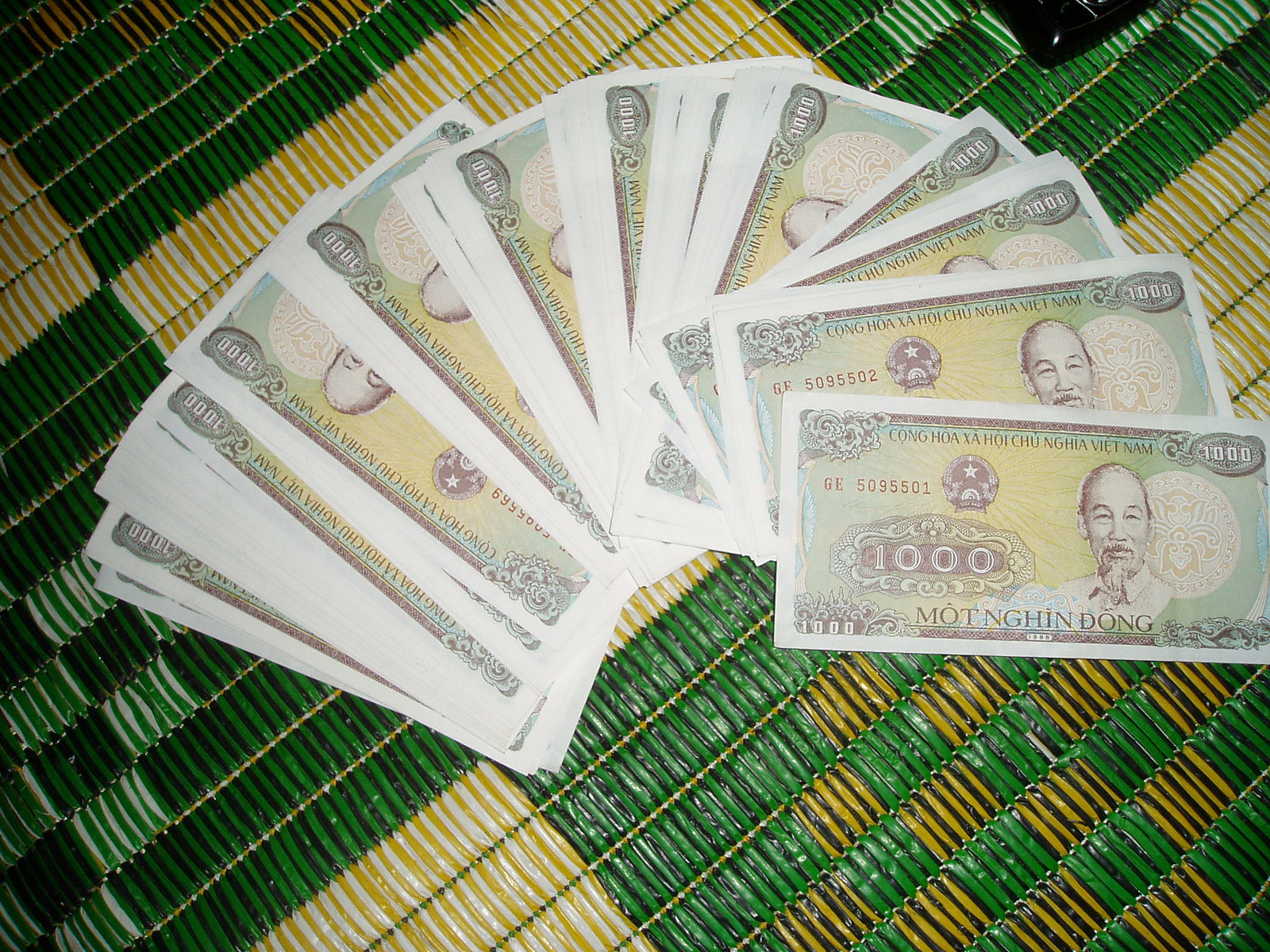The image shows a top-down view of numerous 1,000 Vietnamese Dong notes, fanned out in a crescent shape. These notes, totaling up to around 40, are spread out as if they were playing cards. The currency, predominantly featuring shades of green with hints of blue, yellow, brown, and white trim, showcases a portrait of a man—likely Vietnamese—on the right-hand side of each bill. The entire arrangement of money is laid atop a woven mat, possibly plastic or wicker, adorned with large squares of varying colours, including combinations of green, light green, dark green, yellow, and white. This woven surface may be a table or the base of a chair, and its intricate pattern enhances the detailed and colourful setting of the image.